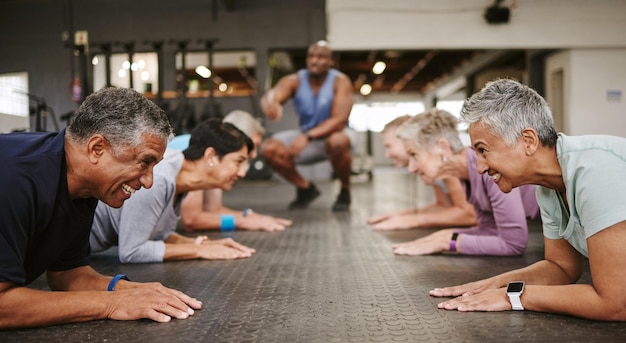In a professional gym setting, six older participants are engaged in a fitness class. They are arranged in two rows, with three people in each row, facing each other on the dark gray floor. All participants are in a plank position, appearing to be mid-exercise. In the background, a trainer with dark skin is crouched down, giving instructions. He is wearing a blue sleeveless tank top, gray shorts, and black shoes. The participants vary in appearance: the man on the left, wearing a dark blue t-shirt and a blue bracelet, has gray hair. Opposite him, a woman with short gray hair wears a light-colored t-shirt and a watch on her left wrist. The other participants are also middle-aged to elderly individuals focused on their workout, with expressions that suggest a mix of concentration and exertion. The atmosphere indicates a professional and guided fitness environment.